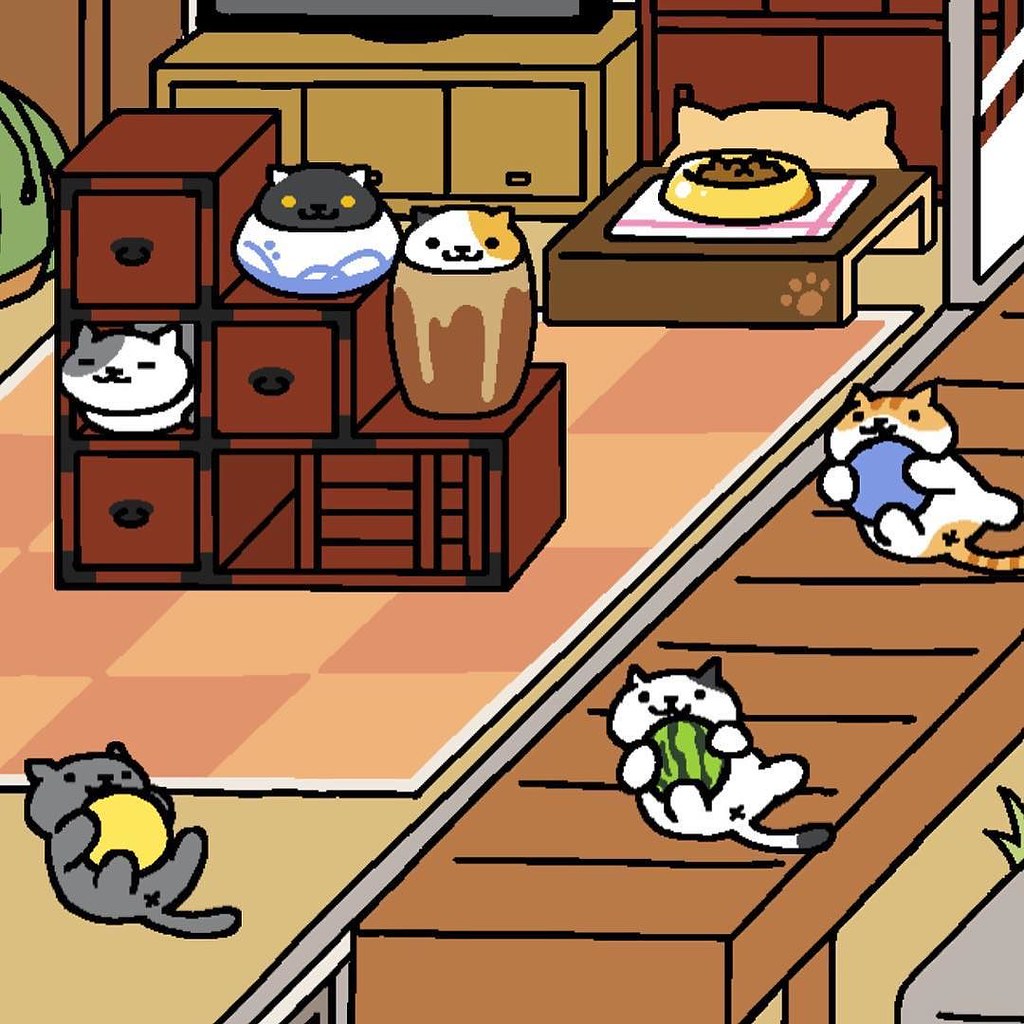In this digital, cartoon-like image resembling a scene from a video game set in a traditional Japanese home with sliding doors, numerous cats are scattered around a room designed to be their playful haven. In the center, three cats lie on their backs, each playfully toying with a colorful ball perched on their tummies: a gray cat with a yellow ball, a white cat with a green striped ball (resembling a watermelon), and a white with orange-striped cat with a blue ball. A distinctive Japanese storage dresser stands in the room, where two cats are nestled comfortably in pots and another peers out from one of the cubbies. The room also features a low table draped with a pink and white tablecloth, hosting a yellow food bowl filled with brown kibble. The room's palette includes hues of brown, medium tan, weathered red, and various shades of green, yellow, blue, and white, capturing a whimsical and cozy atmosphere for the playful felines.